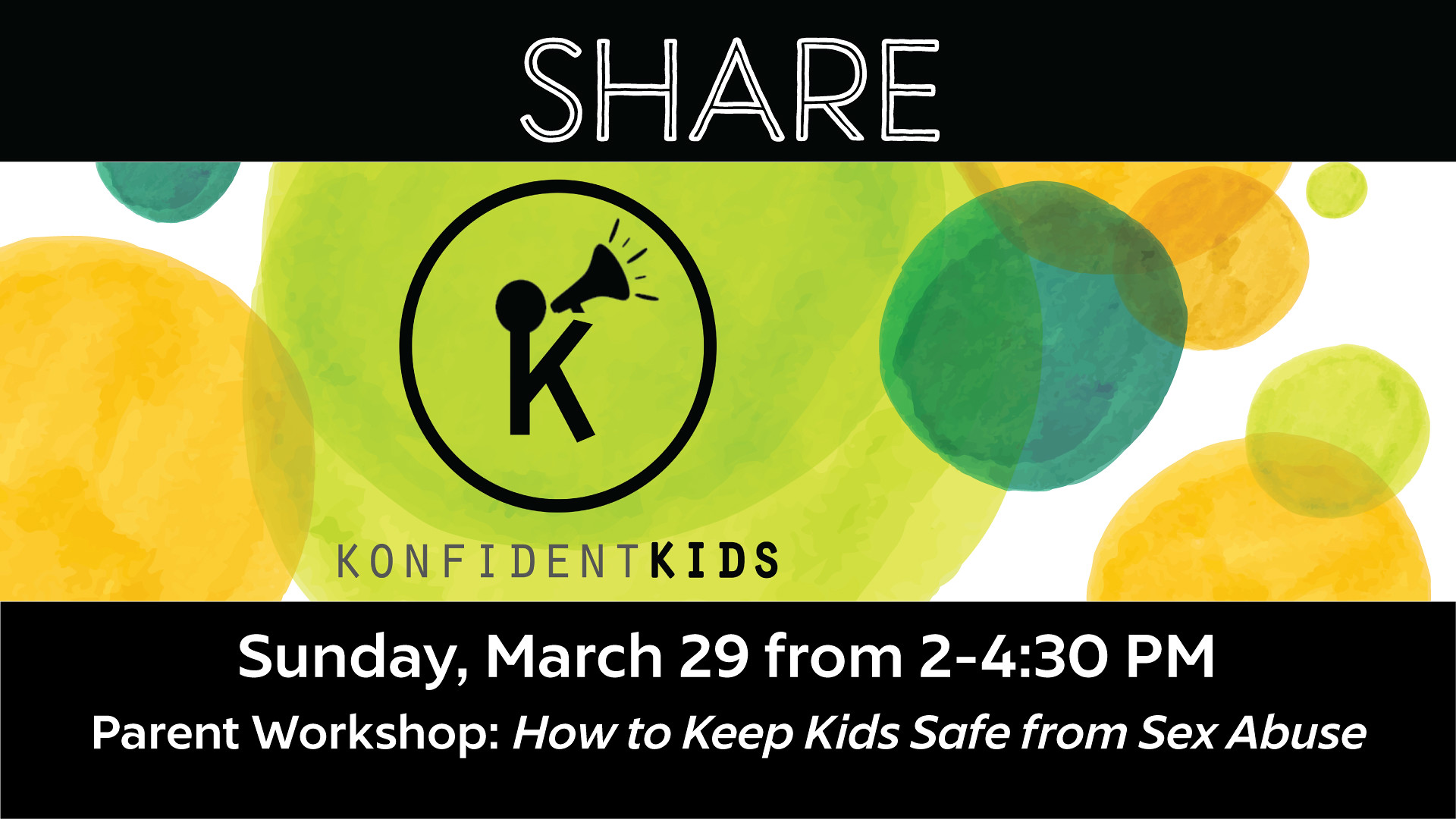The image appears to be a digital advertisement or notification for an upcoming event. It features a black border at both the top and bottom. Centered on the top black border in large white font is the word "SHARE." The bottom black border contains white text that states, "Sunday, March 29th from 2 to 4:30 p.m., Parent Workshop, How to Keep Kids Safe from Sex Abuse."

In the center of the image, a multicolored design features overlapping circles in various shades of yellow, light green, dark green, and a green-blue color, all set against a white background. Prominently displayed within these circles is a black circular logo featuring the letter "K" with a megaphone symbol. Beneath this logo, the words "Confident Kids" appear in black text, drawing attention to the name of the initiative or organization sponsoring the event. The overall layout and the use of colors suggest a focus on creating a visually engaging advertisement for a significant educational workshop aimed at parents.